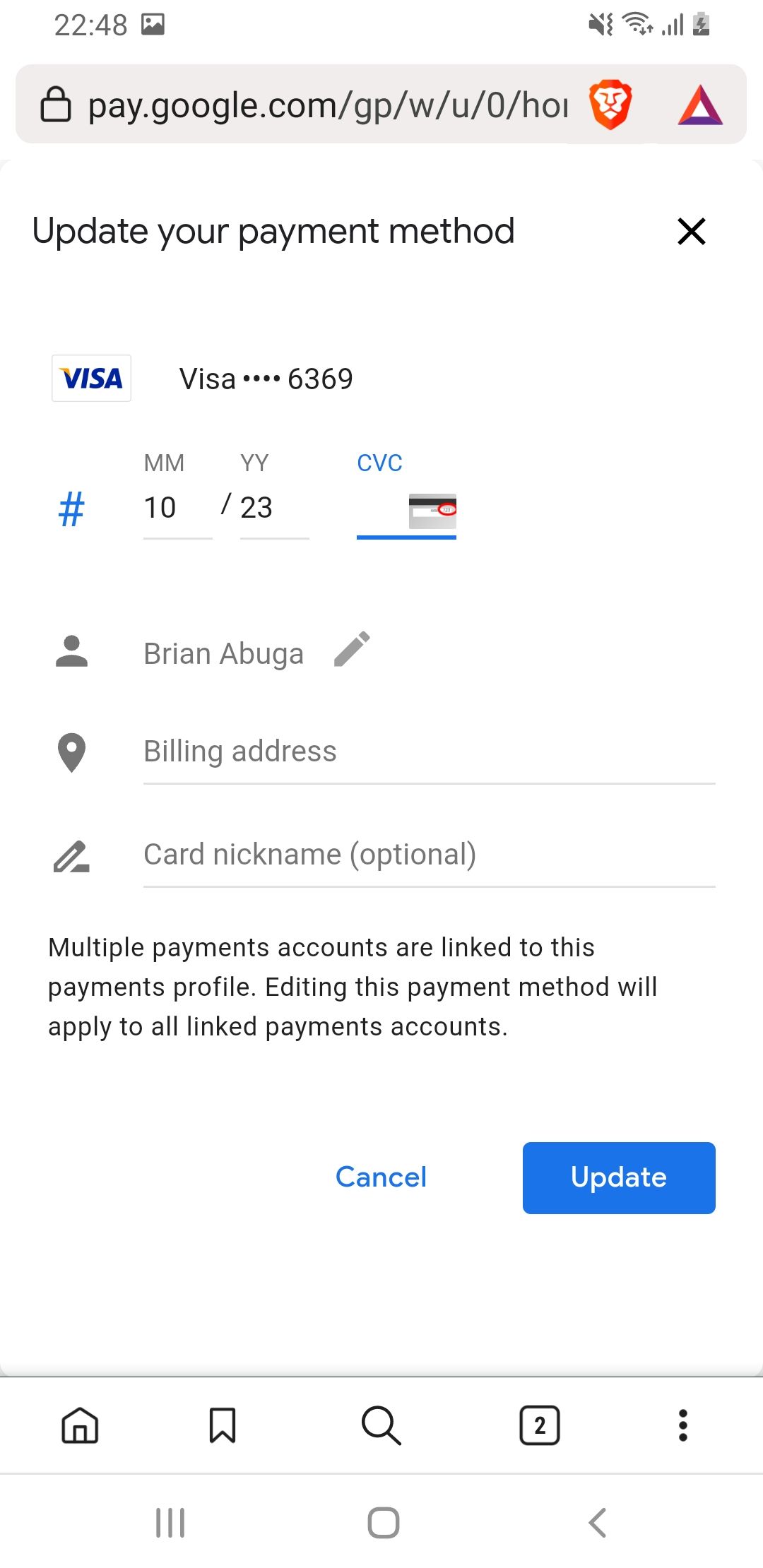**Descriptive Caption:**
A screenshot of a mobile phone displaying the payment method update page on the Google Payments website (pay.google.com). At the top, there is an "X" icon allowing the user to exit the screen. The user is currently updating a Visa card ending in 6369, which expires in October 2023. There is an empty field for entering the CVC code highlighted with a blue underline. Below, the user's name, displayed as "Brian Abuga," can be edited by tapping a pencil icon next to it. Further down, fields for the billing address and an optional card nickname are visible. A message indicates that multiple payment accounts are linked to this payment profile, and any edits will apply to all linked accounts. At the bottom of the screen, there is a blue "Cancel" hyperlink and a blue "Update" button. Navigation options for 'Home,' 'Save,' and 'Search' are presented at the very bottom of the page.